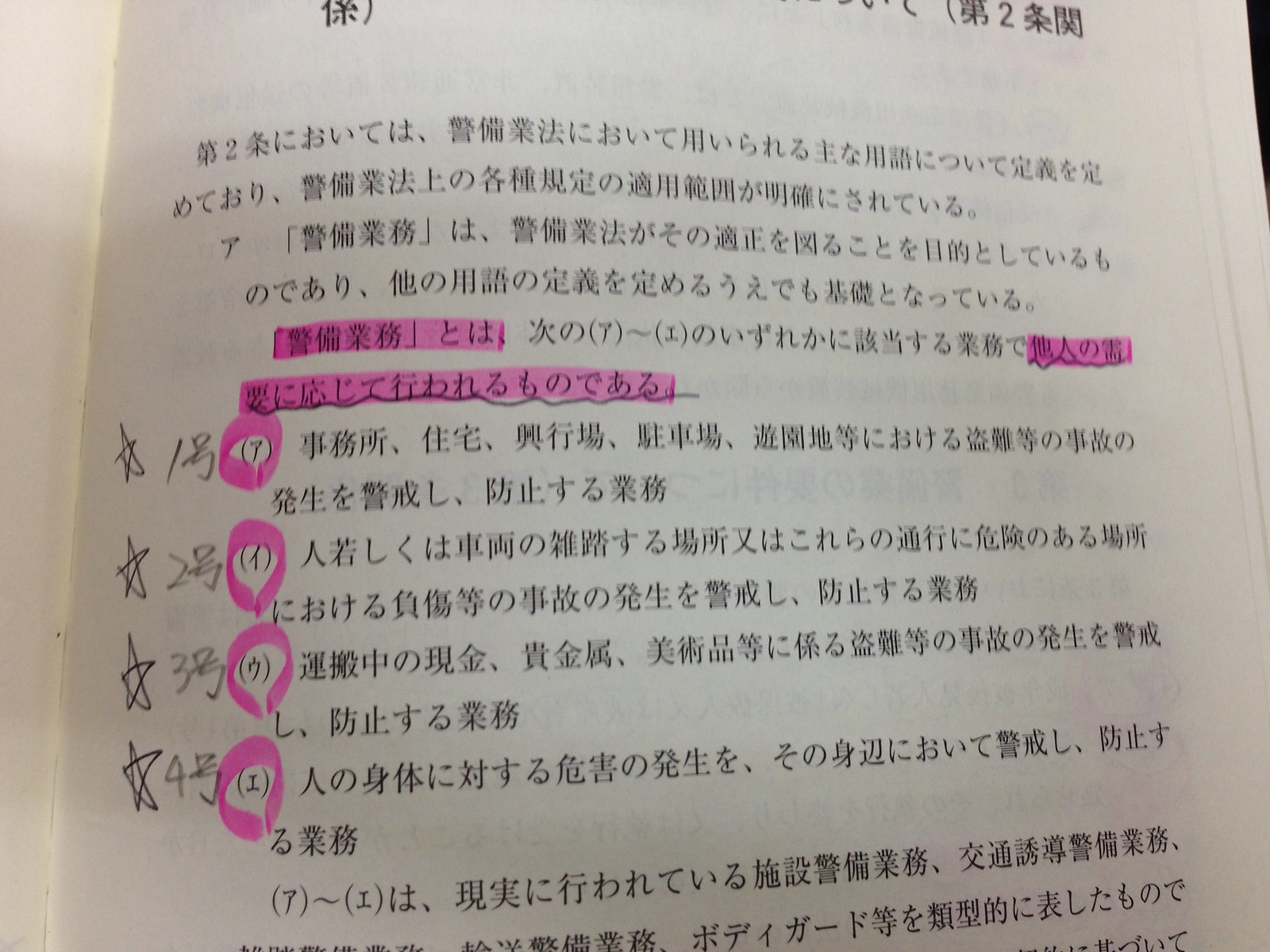This image depicts a close-up view of a formal Asian document printed on white cream paper. The content includes Chinese characters in a black, printed font, suggesting it was created using a computer or electronic device rather than handwritten. Notably, the document features both Asian and American numerals, with the number '2' appearing prominently near the right-hand corner and within the first paragraph.

Distinctive markings are made with a pink highlighter, emphasizing several lines of text and a sequence of four starred and numbered points: 1, 2, 3, and 4. The highlighted sections include half-sentences and individual digits near the stars, which are encircled in pink. The document appears to be well-organized, with the highlighted and circled elements drawing attention to specific details amid the dense Chinese writing.